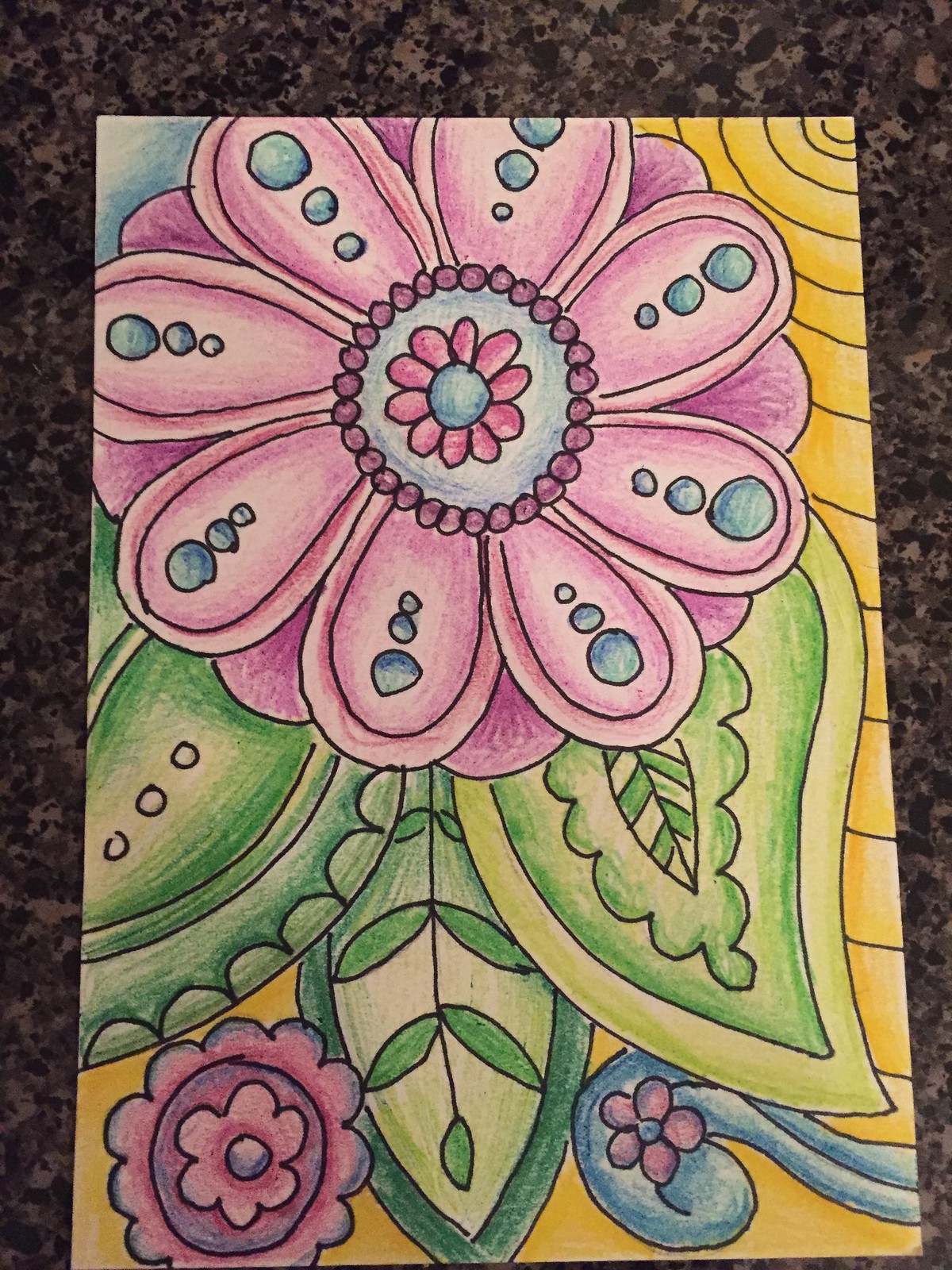The image features a top-down view of a rectangular piece of artwork, most likely a drawing on paper, showcasing a prominent purple flower with thick, rounded petals. Each of these petals is adorned with three blue circles that start small near the center and grow larger towards the edges. The flower's bulb is blue, speckled with purple dots, and has multiple purple shapes extending from it. Surrounding the flower are multiple large green leaves with distinct black ink patterns, each pattern unique to its respective leaf. A smaller purple flower, distinct in that it lacks blue dots, is located at the bottom left of the image. Additionally, another blue petal-like element curves upward from the bottom left to the bottom right. The background surrounding the flower is bright yellow, particularly on the right-hand side and at the bottom of the drawing. This entire artwork is placed on a granite table characterized by a mixture of light tan and black splotches.